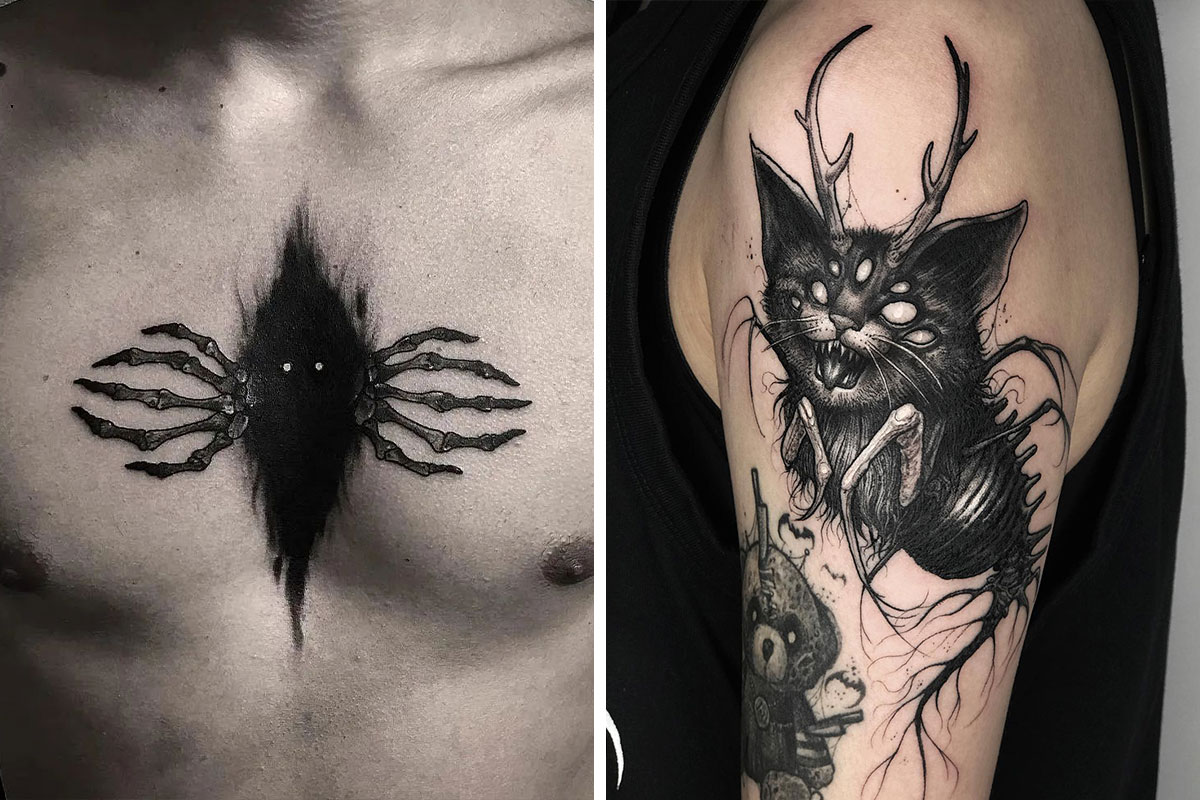This image set features two detailed black and white tattoos on different parts of a man's body. The left image showcases a man's chest with a tattoo of a dark, shadowy figure situated centrally. This demonic figure appears to be oozing like smoke, stretching out with skeletal, claw-like fingers that reach across both sides of his chest, encompassing the nipples. Two ominous black dots serve as the eyes, giving the impression of a creature crawling out from a dark, diamond-shaped void in the middle of his chest.

In the right image, a tattoo spans the man's shoulder and upper arm, depicting a nightmarish cat-like creature. This black cat has bat-like ears, antlers that curve inward at the tips, and at least six eerie eyes scattered across its face. Its mouth is open, revealing sharp fangs, while its front legs resemble those of an insect, complete with long hairs. The spine of the cat transforms into a beetle-like shell with long, hairy strings trailing down. Below this cat-like entity is a disturbing teddy bear tattoo, marred with a knife impaled in its head and wielding a pistol. The entire ensemble of tattoos creates an eerie, grim tableau rendered solely in black ink, standing in stark contrast to the man's light skin.